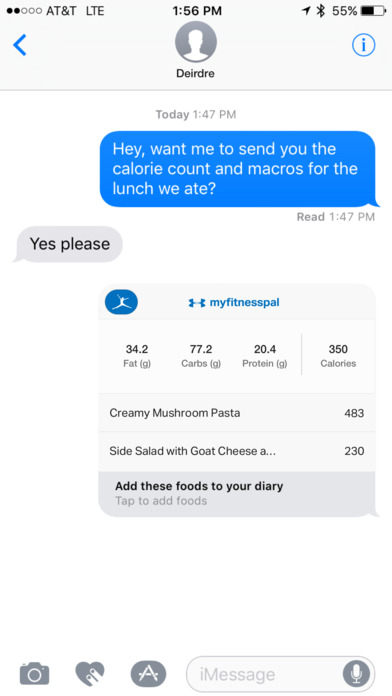This image is a detailed iPhone screenshot capturing an iMessage conversation. At the top of the screen, the status bar displays 2 out of 5 bars for cellular signal strength and AT&T LTE as the internet provider. The current time shown is 1:56 PM. Location services and Bluetooth are active, and the battery is at 55% charge.

The conversation is with a contact named DareJray, whose profile picture is currently blank. The exchange begins at 1:47 PM, when the person taking the screenshot (screenshoter) sends a message saying, "Hey, want me to send you the calorie count and macros for the lunch we ate?" This message is marked as read at 1:47 PM. DareJray responds promptly with, "Yes, please."

Following this, the screenshoter shares a screenshot from the MyFitnessPal app. The app's logo and name are visible, along with nutritional details. The shared nutritional information indicates 34.2 grams of fat, 77.2 grams of carbohydrates, and 20.4 grams of protein, totaling 350 calories. The specifics state that the creamy mushroom pasta contains 483 calories, and the side salad with goat cheese contains an additional 230 calories. However, these calorie counts appear inconsistent with the 350 calories total mentioned.

There's also an option to "Add these foods to your diary," with an instruction to "Tap to add foods."